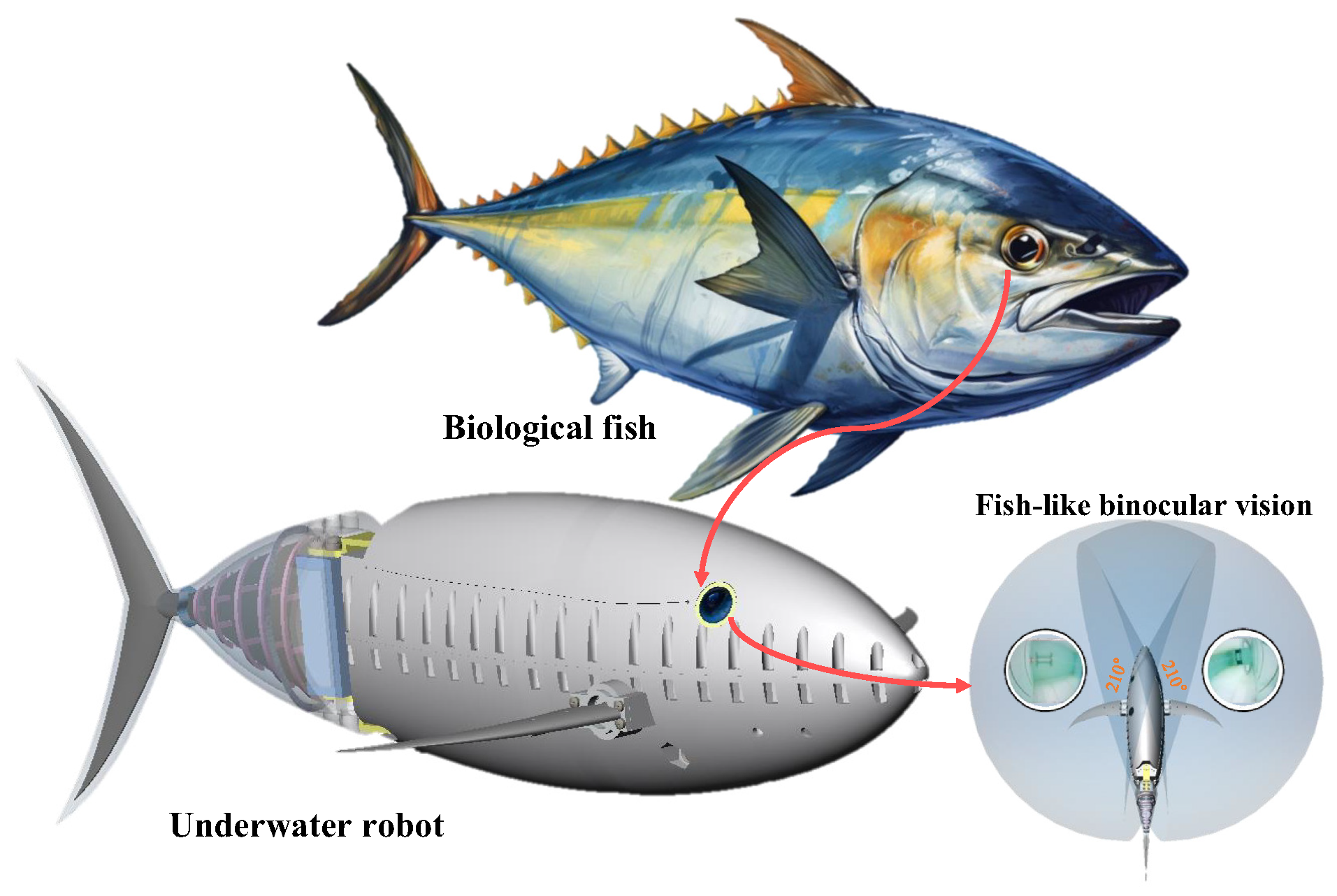This detailed image primarily showcases a comparison between a biological fish, specifically a tuna, and an underwater robot designed to resemble the fish. The illustration style is clean and detailed, set against a simple white background, likely the computer screen.

At the top of the image, a fully colored depiction of a tuna occupies the central position, labeled "biological fish" in black text. This tuna is characterized by a bright blue body with a prominent yellow stripe running along its side. The head is silver with a golden shimmery area behind the eye, which itself has a golden ring and a black center. The dorsal fin is orange, and the tail fins are black and orange, with additional blue and yellow fins along its sides. Yellow spines are visible along the top and bottom of its back end, with blue fins underneath.

Directly below this, on the left, is a robotic counterpart labeled "underwater robot." This robotic fish mimics the shape of the biological tuna but is colored in a metallic silver with blue eyes. Silver fins and blue-silver strips run down its sides, and the inner workings of the tail are highlighted with pink rings.

To the right, a visual representation of the "fish-like binocular vision" is provided, illustrating how the underwater robot can see in a manner similar to the biological fish. An arrow connects the biological fish to the robotic version, emphasizing their resemblance in both form and function. Overall, the image highlights the similarities and technological mimicry involved in the design of the underwater robot in contrast to the natural anatomy of the tuna.